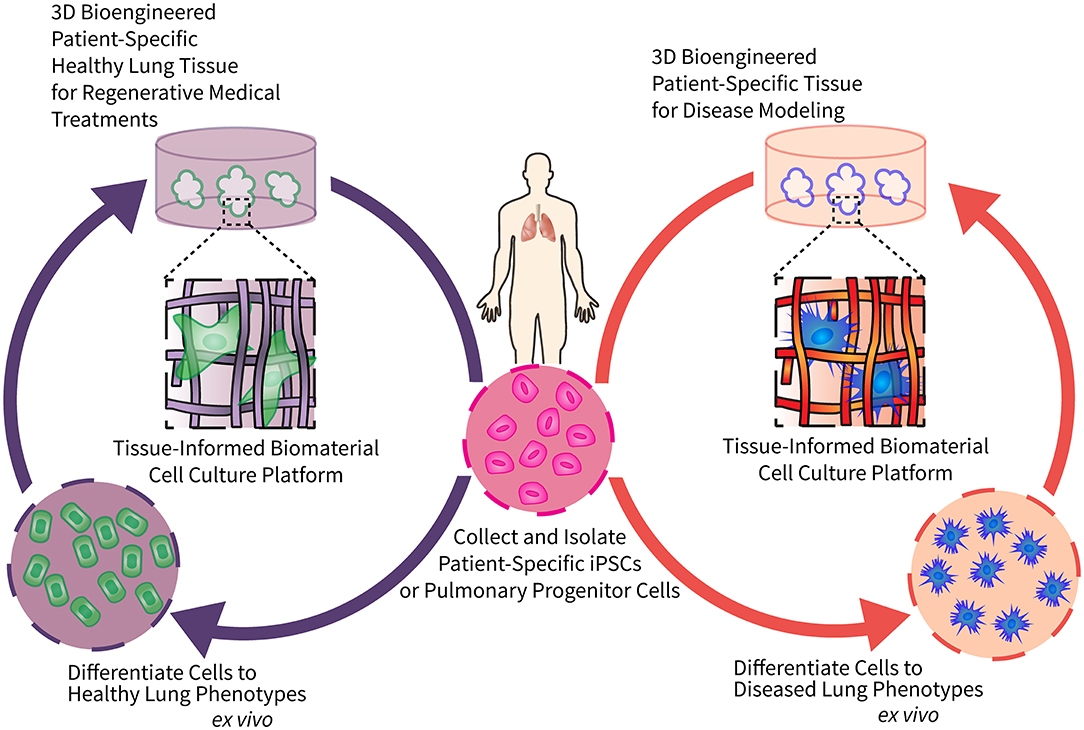The diagram is a detailed illustration of a biotechnological process involving 3D bioengineered lung tissue tailored to individual patients for both regenerative medical treatments and disease modeling. It features two circular, cyclical sections: the left circle is purple and titled "3D Bioengineered Patient-Specific Healthy Lung Tissue for Regenerative Medical Treatments," while the right circle is red, titled "3D Bioengineered Patient-Specific Tissue for Disease Modeling." Central to the diagram is a simplified illustration of a person, highlighting their lungs.

Beneath the person is a smaller pink circle representing cells, with the label "Collect and Isolate Patient-Specific iPSCs or Pulmonary Progenitor Cells." Each circular process also prominently displays the term "Tissue-Informed Biomaterial Cell Culture Platform" at its center. The purple circle on the left includes details on differentiating cells to healthy lung phenotypes, ex vivo. Conversely, the red circle on the right details differentiating cells to diseased lung phenotypes, ex vivo. The diagram effectively uses color-coding and cyclical arrows to delineate these complex bioprocesses, emphasizing the collection, differentiation, and application of patient-specific cells in lung tissue engineering.